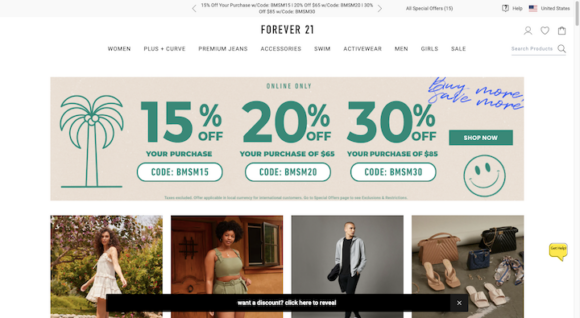This horizontally-oriented image, captured from the Forever 21 website, provides a typical view for desktop or smartphone users. At the top of the page, there is a thin gray strip displaying promotional information about various discount offers. Accompanying this strip, a series of icons and links are visible: to the right, it reads "All Special Offers" and includes a "Help" button, the American flag, and the text "United States."

Directly below this gray strip, the background transitions into plain white, reminiscent of a typical computer screen. Prominently centered in uppercase letters is the "FOREVER 21" logo. Below the logo, a series of clickable options are available, categorized as Women, Plus and Curve, Premium Jeans, Accessories, Swim, Activewear, Men, Girls, and Sale. Further to the right, additional icons include a user profile, a heart for wishlist items, a shopping bag for the cart, and a search icon for products. These are followed by promotional messages depicting discount tiers: 15%, 20%, and 30% off based on purchase levels, which are denoted as online-only offers and highlighted in blue with the slogan "BUY MORE SAVE MORE." A "Shop Now" button with a smiley face directs users to start shopping.

Below the promotional banners, there appears to be a series of clickable images showcasing different people modeling clothing, shoes, and accessories. A black bar crosses the bottom portion of these images, featuring a call-to-action: "Want a Discount? Click Here to Reveal."

This comprehensive layout is common for e-commerce sites, aiming to provide users with quick access to product categories, promotional offers, and personalized account features.